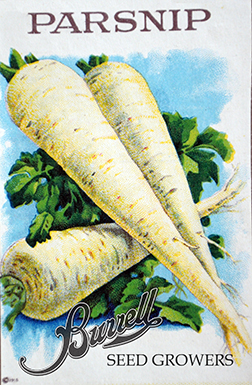This image is a photograph of an old-fashioned seed packet for parsnips. The packet itself is predominantly white with a decorative blue sky background in the center and features a collection of three parsnips surrounded by green leaves. Specifically, one large parsnip is laid horizontally with its root end to the right side, while two additional parsnips lie diagonally across it, with their thicker ends pointing toward the upper left corner and their tapering root ends toward the lower right. Notably, the parsnips are depicted with a slight yellowish hue, enhancing their realistic appearance against the painted foliage.

At the top of the seed packet, the word "PARSNIP" is prominently displayed in large, dark purple, all-caps text with a hand-painted aesthetic. The bottom of the packet features the name "Burrell" in cursive, followed by "SEED GROWERS" in black, uppercase text, suggesting the manufacturer's classic branding style. This vintage illustration embodies the detailed and artistic approach traditionally used for seed packaging.